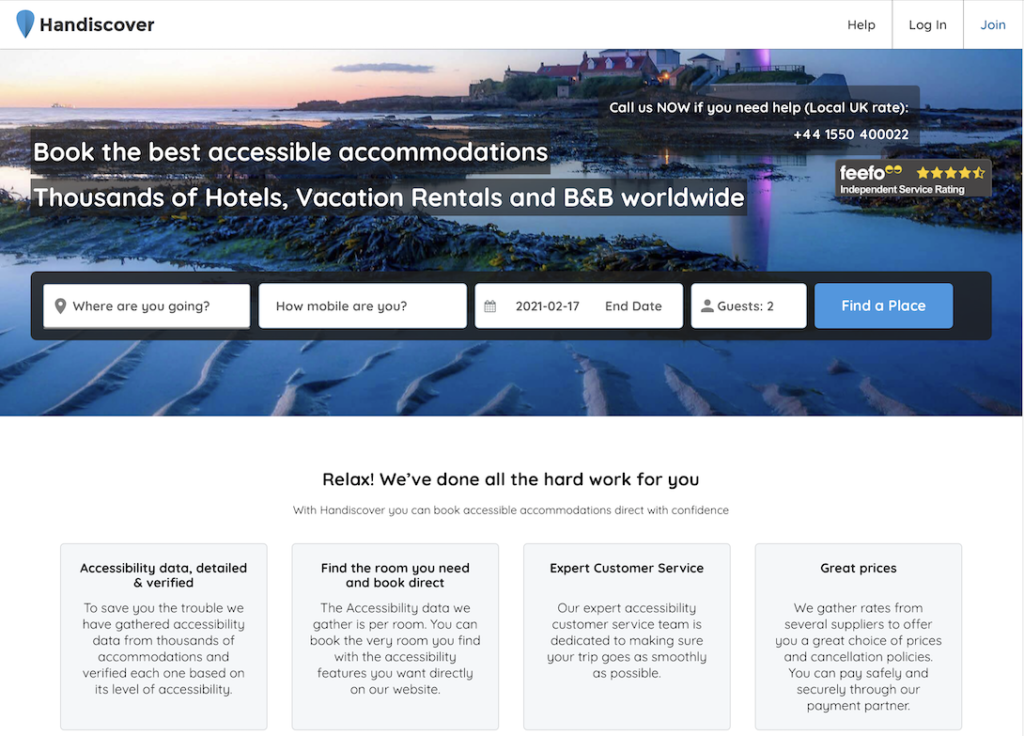The image is a detailed promotional banner for "Handiscover," featuring a structured and visually appealing layout.

**Upper Section Description:**
- **Header:** At the very top, a white rectangular header spans the width of the image, bordered in light gray. In the upper left corner, the logo and name "Handiscover" are displayed. The logo resembles a stretched, shield-like guitar pick in light to medium blue. The name "Handiscover" is written in bold, initial capital black font. To the far right of the header, three options—"Help," "Login," and "Join"—are separated by vertical black lines, with "Join" positioned at the outermost right.

**Main Image Description:**
- **Background Image:** Below the header, a landscape image captures a tranquil seaside resort scene at sunset. The horizon glows in hues of orange and yellow, complementing the distant buildings and calm water in the foreground.
- **Overlay Text:** Against this scenic backdrop, promotional text is displayed within contrasting dark gray and white boxes:
  - **Left Side Text:** 
    - "Book the best accessible accommodations" (in white text within a dark gray box).
    - "Thousands of hotels, vacation rentals and B&B worldwide" (in white text within a dark gray box just below the first line).
  - **Center Text:**
    - A small white rectangular box contains "FEEFO," along with a 4.5 out of 5-star rating depicted with yellow-orange stars, followed by "Independent service rating."
  - **Lower Overlay Text:**
    - A black horizontal box split into five sections:
      1. **"Where are you going?"** featuring a pin drop icon.
      2. **"How mobile are you?"**
      3. **Start and end dates with a calendar icon:** Displayed as "2021-02-17" and "End date."
      4. **"Guests 2"** with a head-and-shoulders icon, indicating two guests.
      5. **"Find a place"** in white text on a blue background, functioning as a call-to-action button.

**Lower Section Description:**
- **Text Block:** The bottom half of the image features a white background filled with descriptive text:
  - **Centered Header:** "Relax! We've done all the hard work for you."
  - **Subheader:** "With Handiscover, you can book accessible accommodations direct with confidence."
- **Information Boxes:** Below this, four light gray square boxes are aligned horizontally, each with centered headers and text:
  1. **"Accessibility data, detailed & verified"**
  2. **"Find the room you need and book direct"**
  3. **"Expert customer service"** (with "E," "C," and "S" capitalized).
  4. **"Great prices"** (with "G" capitalized).

Each square box contains several lines of additional centered, justified text, detailing the benefits and features of using the Handiscover service to find accessible accommodations.